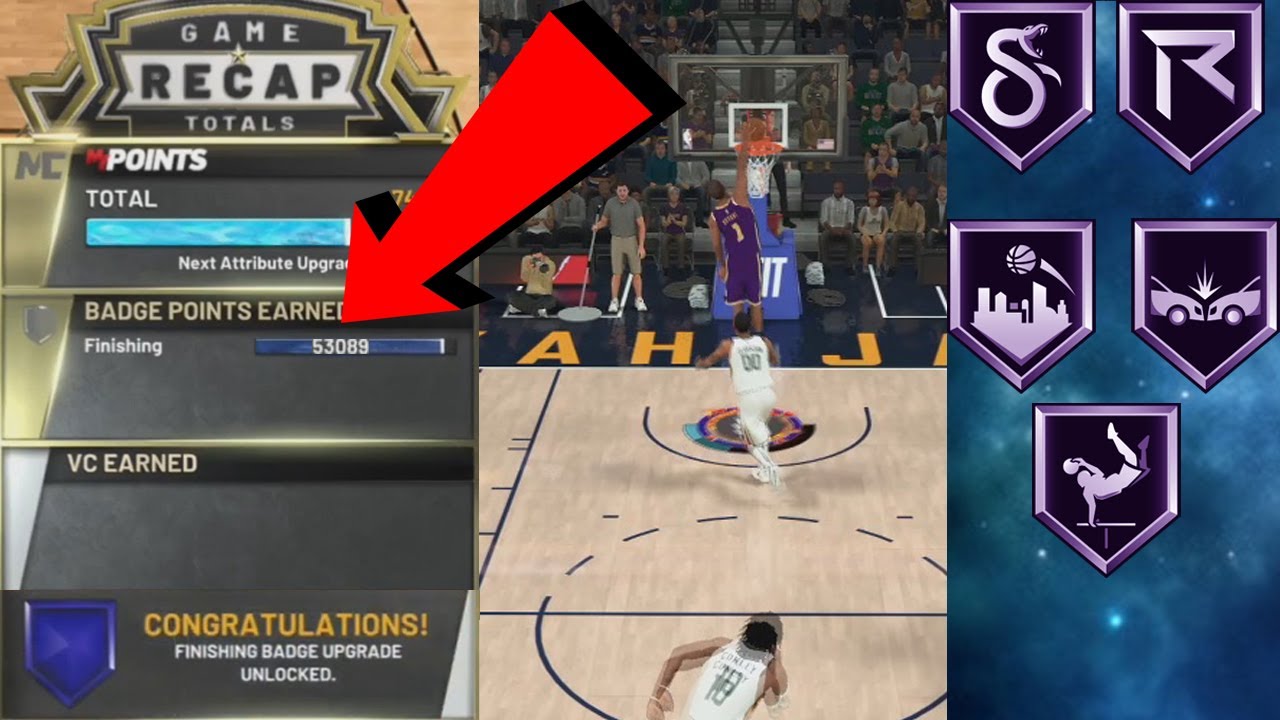This caption has been formulated and cleaned up to provide a detailed description of the images:

The image is a composite of three vertical screenshots arranged horizontally. The first screenshot appears to be from a video game user interface displaying "Game Recap Totals" at the top. This UI is divided into three black panels separated by shining gold borders, each with its own header: "Points," "Badge Points Earned," and "VC Earned." At the very bottom, there is another panel without a gold border that features a blue polygonal badge with gold text saying "Congratulations" and white text below stating "Finishing Badge Upgrade Unlocked."

The center screenshot is an in-game scene from a basketball video game. It shows two basketball players in white jerseys with green text, running towards an opposing player who is executing a slam dunk. The dunking player is wearing a purple jersey with yellow numbers and trim. The background features a virtual crowd behind the basketball hoop.

The third screenshot contains three rows of different icons, all sharing a similar polygonal aesthetic. These icons are square at the top and taper to a diamond point at the bottom, with a purple metallic finish and black interiors featuring metallic icons. The background of this screenshot is a blue nebula.